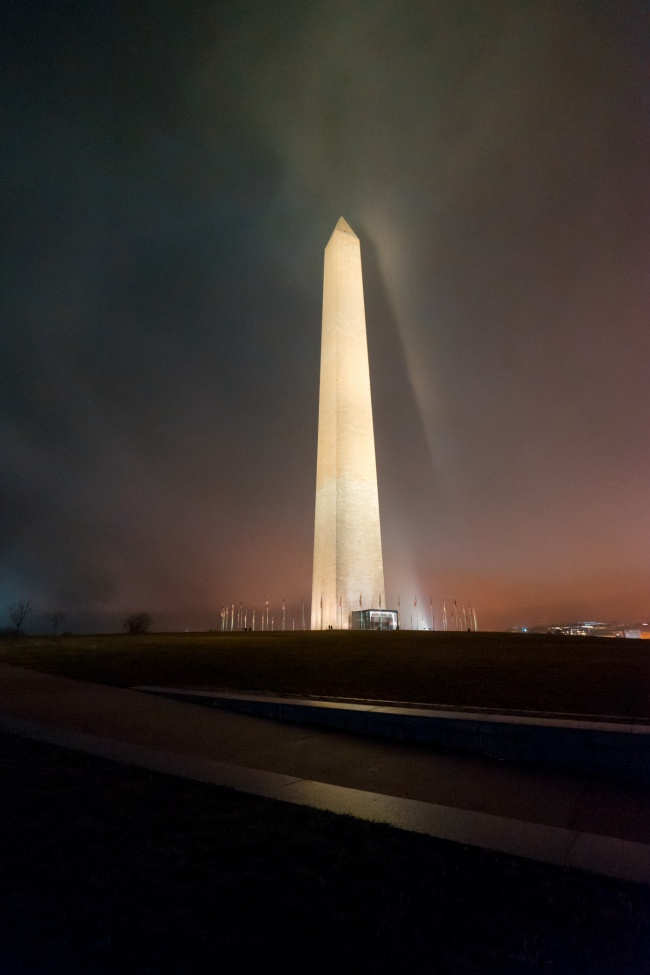This is a detailed nighttime image of the Washington Monument. The monument stands prominently, illuminated in white and cream lights that extend up into a dark sky, which shows a gradient of black transitioning to orange near the horizon. The photograph is taken from a slightly lower perspective, making the towering structure even more imposing. Surrounding the monument is a ring of flagpoles, each bearing the United States flag, although their colors are indistinct due to distance. In the foreground, a patch of grass leads up to hedges and additional greenery, including bushes and trees with brown stems. To the lower left, there is a street and a gray sidewalk with a white dividing line, accompanied by a slanted ledge. Additionally, the lower portion of the monument shows a bus, potentially a tourist bus, that appears to be leaving the scene. On the right side of the image, a nearby structure—possibly the Pentagon—appears lit up and is about three or four stories high. In the distant background, there are more lights, hinting at the presence of a city area. The overall ambiance of the picture is serene and majestic, with the monumental edifice dominating the view.